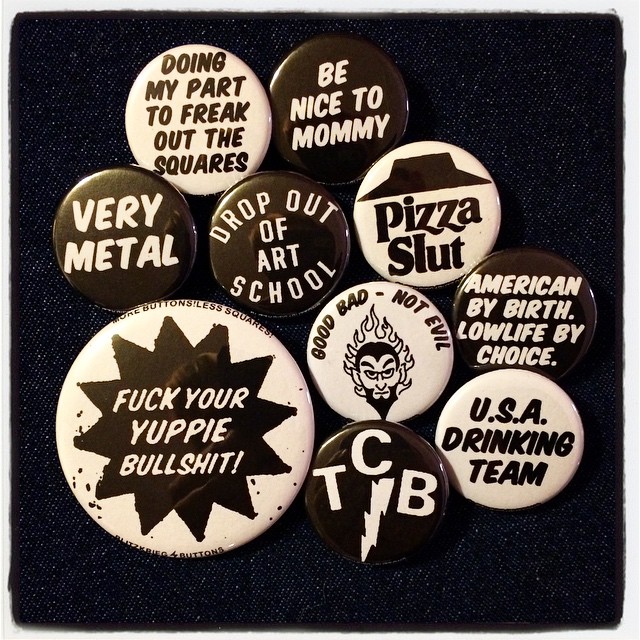The image depicts a display of vintage buttons arranged in a circular pattern on a black felt background. All the buttons are round and primarily feature black and white designs. Starting from the top left, the first button has a white background with dark print, stating "Doing my part to freak out the squares." To its right, a dark button with white print reads "Be nice to mommy." In the next row, the leftmost dark button with white lettering says "Very metal," followed by another dark button with the inscription "Drop out of art school." Further right is a white button with dark elements mimicking the Pizza Hut logo but reading "Pizza Slut." The third row starts with the largest button on the left, which is white with a jagged-edged black shape in the center, reading "Fuck your yuppie bullshit." To its right is a small dark button with a white lightning bolt and the letters "TCB" above it. The farthest right button in this row is white with black lettering, stating "USA Drinking Team." Among other buttons, there’s one with a devil image and the words "Good, Bad, Not Evil," and another that reads "American by birth, low life by choice." The overall aesthetic is predominantly black and white with some sepia tones, and many of the buttons feature provocative or humorous messages.